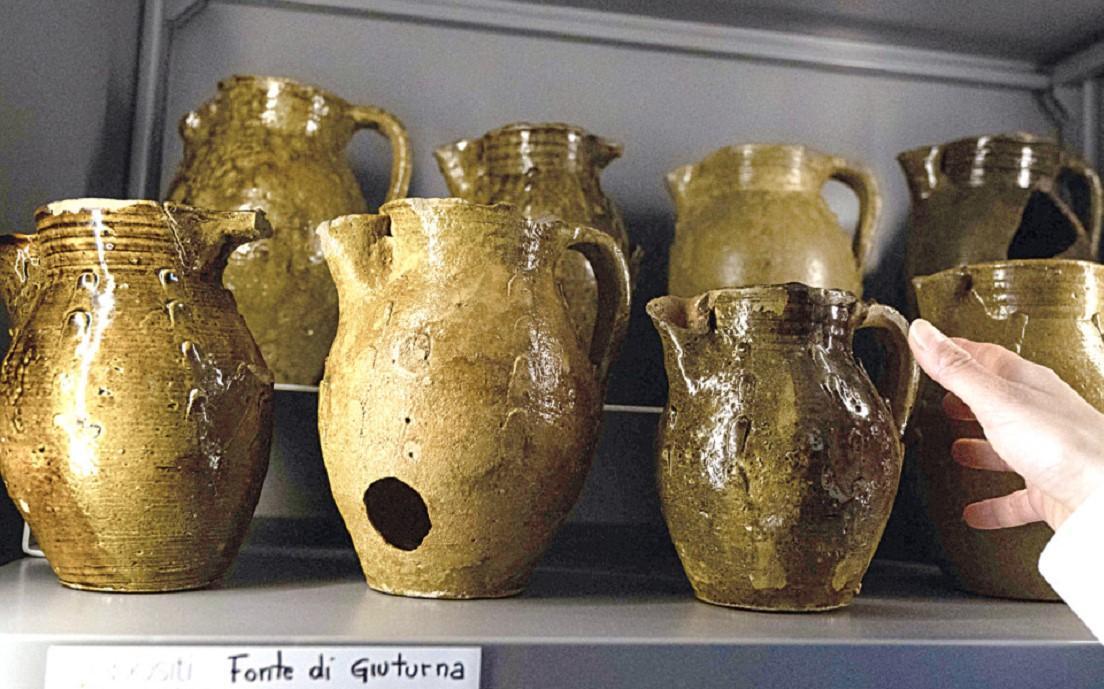The image features a collection of eight green vases arranged on a gray metal shelf. Four vases are positioned in the front row, while the remaining four form a line in the back. Each vase appears to vary slightly in its sheen, with a few exhibiting a shinier finish compared to the others. Notably, four of the vases have handles; however, the handles on two of these vases appear to be broken. The meticulous alignment and the contrast between the metal shelf and the vibrant green vases draw attention to the subtle differences in their appearance and condition.